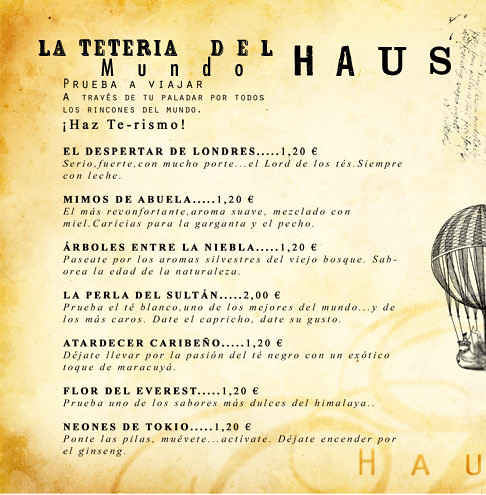This detailed image depicts a textured, yellowish-brown drink menu from a Mexican restaurant, titled "La Teteria del Mundo House." The semi-cursive heading "Preva a Viajar!" is legibly displayed underneath. On the right side, a half-cropped sketch of a hot air balloon, featuring two people, adds a whimsical touch. Decorative curves embellish the background, and faint, illegible handwriting adorns the top. Prices on the menu range from 1.20 to 2 euros, indicating affordable options. Notable items listed include "El Desparto de Londres," "Mimos de Abuelo," and "Arbos entre la Niebla," each priced at 1.20 euros. The bottom right corner features the letters "HAU."